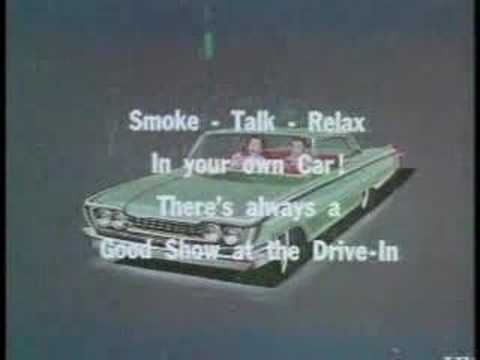This grainy, vintage advertisement—likely from the 1940s or 1950s—features a pale mint green retro sedan, possibly a 1950s Chevy, with two people, a man and a woman, seated inside. The image, which appears to have been photographed from a screen, has a muddy, gray-brown background with a thin black border on the left and right sides. Over the center of the image, white text enthusiastically proclaims: "Smoke - Talk - Relax in your own car! There's always a good show at the drive-in." Despite numerous visual artifacts, the nostalgia and charm of the drive-in era are vividly captured in this classic ad.